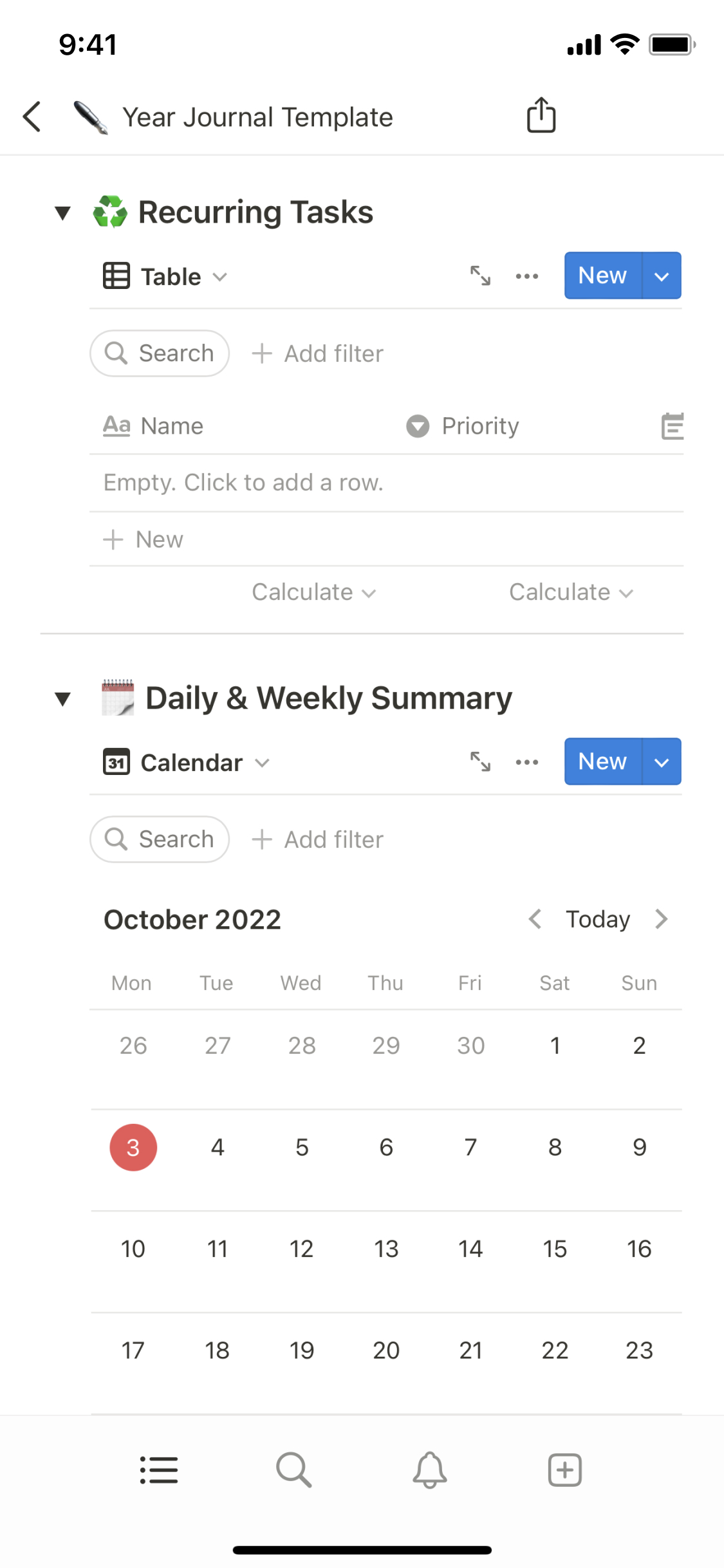This image depicts a detailed view of a cell phone screen showcasing a web page or app interface. At the top of the screen, the status bar indicates a time of 9:41 AM. The phone is fully connected with four bars of signal strength, Wi-Fi enabled, and displaying a fully charged battery icon. The background is predominantly white, providing a clean and clear presentation.

The main content displayed is a "Year Journal Template." The first section is labeled "Recurring Tasks," which offers options to "Add a table," "Search," or "Add filter." You can also input task details such as name, priority, and other specifics, aiding in the management and entry of recurring tasks.

Beneath this section is a "Daily and Weekly Summary," adjacent to a button labeled "Calendar" and a "New" button. Under this, "Search" and "Add filter" options are also available. Highlighted in bold is the date "October 22," with a "Today" marker beside it.

The calendar displayed shows the current date as October 3, 2022. The calendar view begins with the end of September, starting from Monday the 26th through Friday the 30th, followed by Saturday, October 1st. It continues in this format up until Sunday, October 23rd.

At the bottom of the screen are navigation icons including three dots with lines, a magnifying glass for search functions, a bell for notifications, and a plus sign for adding new items, providing easy access to additional features.